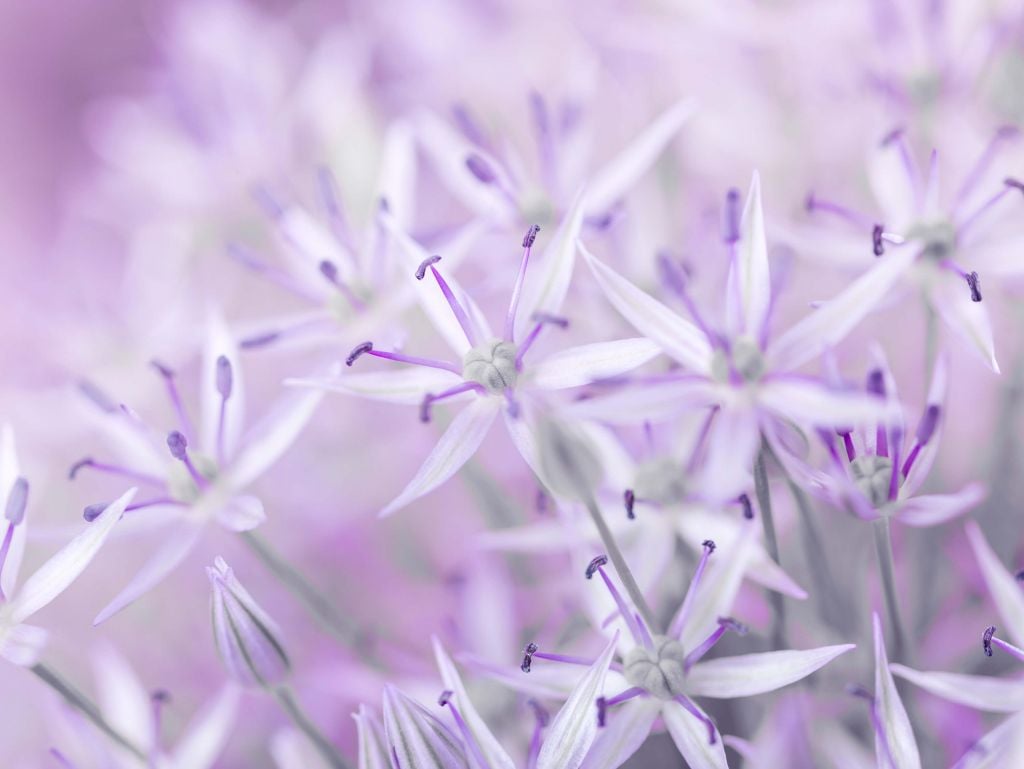This is a detailed close-up photograph capturing a large group of white and purple flowers, approximately 20 or more in total. Each flower showcases six very narrow, long petals. At the center of each flower, there is a round, pumpkin-shaped structure that is predominantly white with hints of green, out of which radiate five pistils and six stamens. The stamens are white with purple tips and have small protrusions at their ends, likely where the pollen is located. The green stems of the flowers are straight and may appear slightly fuzzy. While some flowers remain closed, particularly in the bottom left-hand corner, the majority are fully opened, splaying wide. The photograph primarily focuses on a few flowers in the foreground, leaving the background blurred and adding a lavender hue over the entire image.